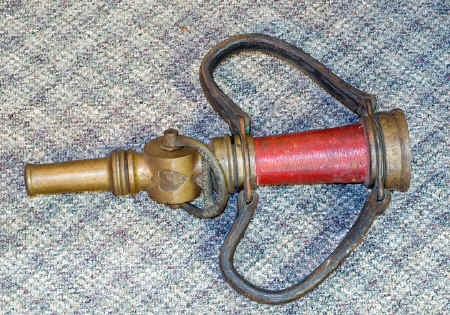The image depicts a detailed close-up of a vintage brass or copper fire hose nozzle, photographed against a patterned carpet. The carpet features light gray diamond shapes that transition from darker gray in the upper right corner to a lighter gray with a brownish hue towards the left. The nozzle itself is a complex piece of apparatus with several distinct components: 

- On the left, there is a small cylindrical section, lighter brown in color, designed to attach to a hose.
- Moving right, the cylindrical part leads to a ring that rises from the top and curves down, possibly serving as a grip or a pressure guide.
- The central part of the nozzle is painted red and flanked by two large, flexible metal handles that extend horizontally on either side, resembling ears.
- Finally, the nozzle flares out again, culminating in an end section where water exits, also made of brass or copper. 

A small curved lever, possibly for adjusting the spray or shutting off the flow, is situated between the red central section and the water exit part. This intricate design hints at its use for controlling and directing high-pressure water flow, likely from a fire hose, offering a glimpse into its robust and functional engineering.